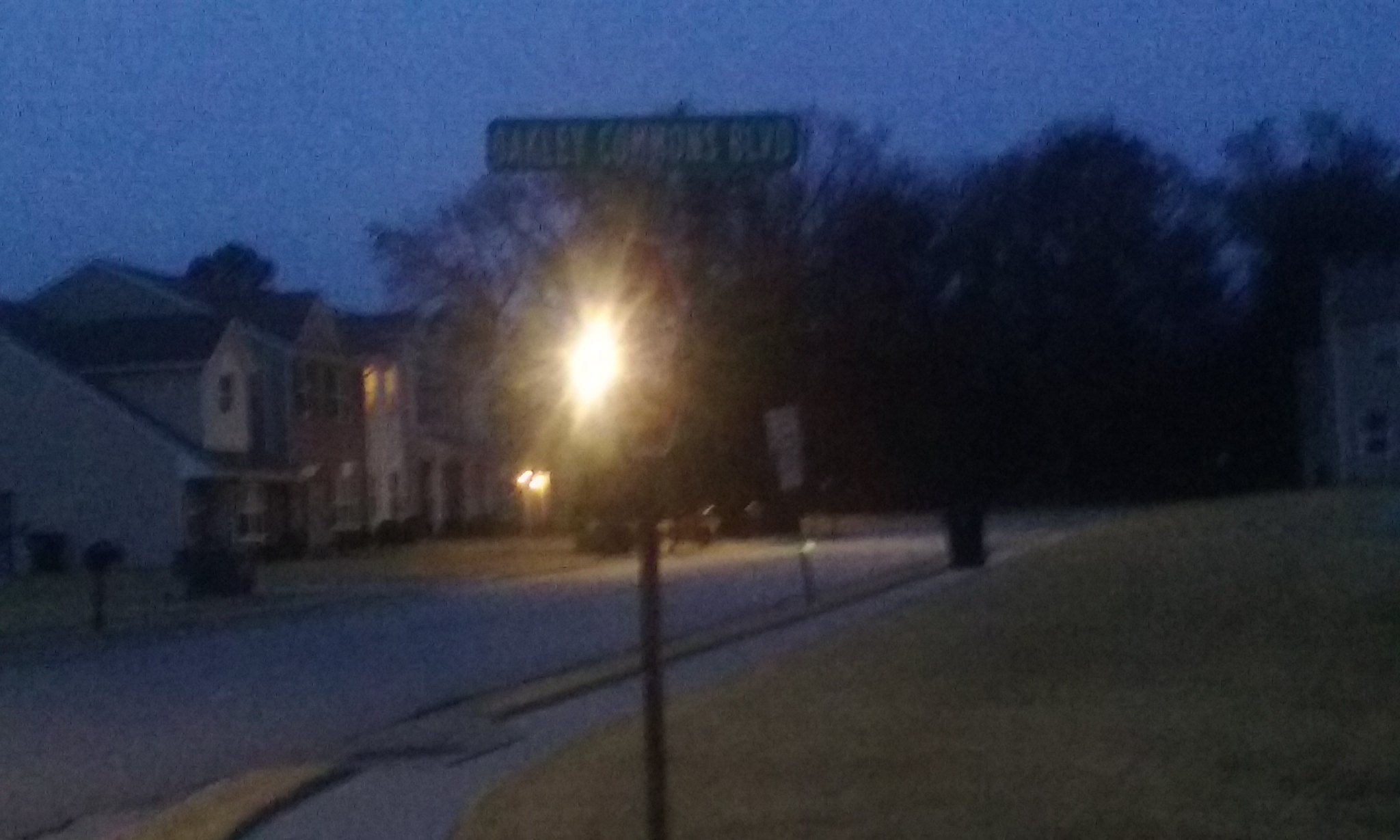The focal point of this slightly blurry image is a stop sign mounted on a small metal pole, positioned at a slanted angle. Above the stop sign, there is a long, green street sign that reads "Barkley Common Boulevard." The scene is set within a neighborhood backdrop, showcasing large houses on the left side of the image, painted in shades of white and light brown. On the right side, a hint of another large house is visible. The background features an expanse of dark, towering trees. The lower portion of the image reveals a road stretching from the bottom left corner into the distance on the right side. Adjacent to the right of this road is a grass field.